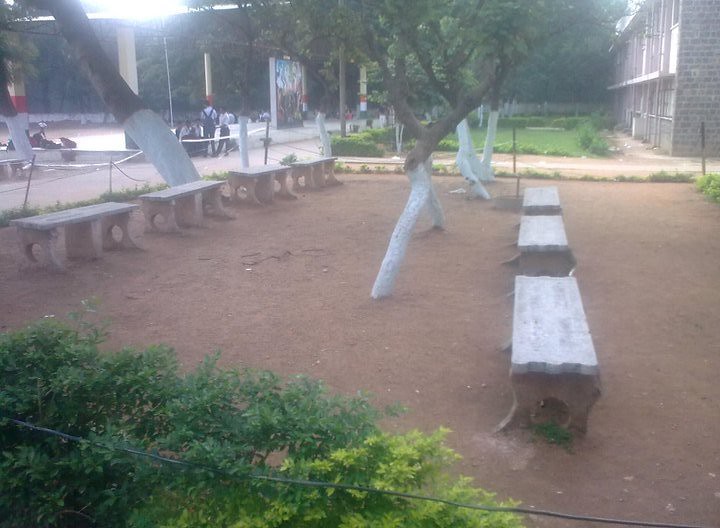The photograph captures an outdoor courtyard, likely part of a school, with a sandy dirt surface and multiple concrete benches with white tops and red bases. The courtyard has seven benches in total, four on the left and three on the right, interspersed with trees that have their trunks painted white. The area appears to be overexposed due to bright sunlight from the top left, and the overall photo quality is amateur.

In the middle distance, to the left of the frame, students with backpacks congregate on a cemented area, possibly a physical education zone. In the background, there is a lawn leading up to a red-brick or grey-brick building, identified as a schoolhouse. The right side of the image shows the school building in more detail, alongside a possible soccer field or court area.

Additionally, there's a wall with a mural or graffiti further in the background. The trees in the courtyard are uniquely twisted, and some foliage is visible towards the left part of the image. The courtyard itself is empty, emphasizing the stark contrast with the lively student area further back.